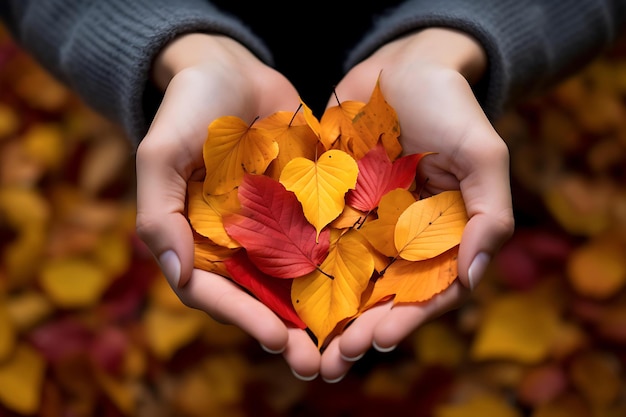The image is an outdoor, autumn-themed photograph focusing on a woman's hands, which are cupped together, forming a heart-like shape with the sides of the palms touching. Her hands are well-manicured with slightly long fingernails adorned with light-colored nail polish. She is wearing a long-sleeved dark gray sweater. The palms of her hands are filled with numerous fall leaves in vibrant colors, including yellows, reds, and oranges, with varying shapes such as rounded, pointy leaves, and traditional maple leaves with three points. A particularly heart-shaped yellow leaf is prominently placed in the center. The background is blurred but showcases a floor covered with an assortment of fallen autumn leaves that mirror the ones in her hands. The image has a sharp focus on the hands and the colorful foliage they hold.